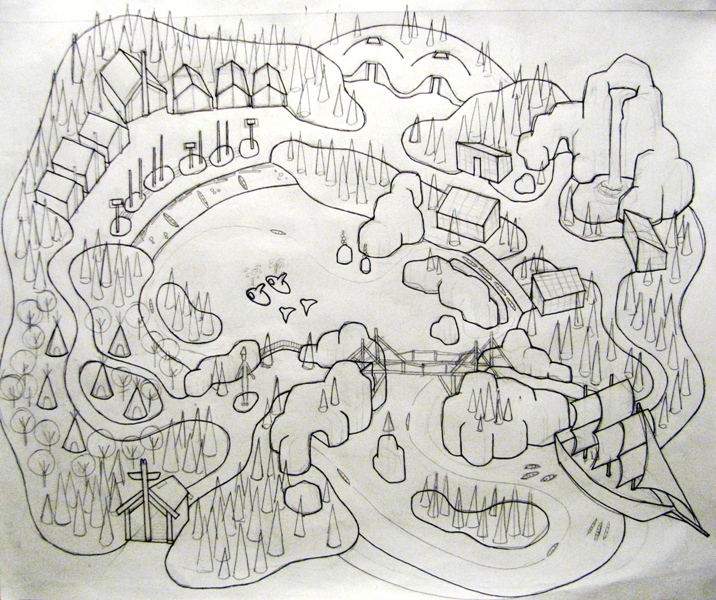This detailed black-and-white drawing, likely created by children, depicts a top-down view of a village nestled in diverse landscapes. At the center, a pond teems with fish, dolphins, and seagulls, hinting at a connection to the ocean. The surrounding area is dotted with conical and round trees, some with a central stem, creating a lush, yet varied terrain. Numerous huts, small houses, and buildings are scattered throughout the village, with silhouettes of more structures, including a church with a cross, visible in various corners.

On the right side of the drawing, a waterfall cascades down from what appears to be a mountain or possibly an artificial structure, complemented by other mountains in the area. A sizeable sailboat with multiple masts is depicted sailing from the right center towards the lower left corner, adding a dynamic element to the scene. Stones are sporadically placed on the ground, enhancing the natural feel of the drawing. The upper center features a whimsical sun with two eyes and rays extending from it, rising amidst silhouettes of clouds and more buildings. Overall, this intricately detailed village map is rendered solely in black lines with gray shading on white paper, capturing the imagination through its simple yet expressive forms.